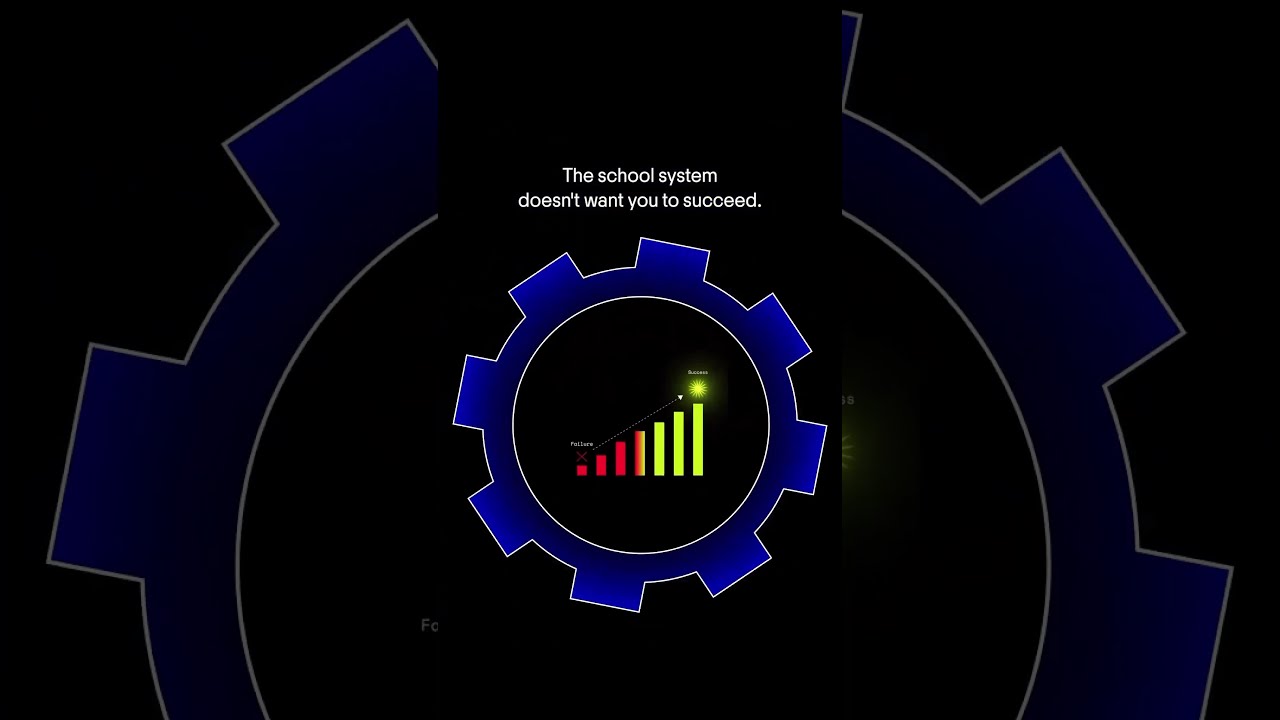The image is a horizontally rectangular graphic divided into three vertical sections. The first and third sections feature darkened close-ups of the central section. The central section showcases a digital illustration against a solid black background. This illustration includes a prominent blue cog or gear with notches around its circumference, set in front of a darker blue, larger cog in the background, creating a layered depth effect. 

In the middle of the blue gear, there's a bar graph with bars increasing in height from left to right. The lower bars are red, transitioning to yellow as they get higher, with an arrow starting at the lowest red bar and pointing to the highest yellow bar. 

Above the gear, centered text in small white print reads, "The school system doesn't want you to succeed." This stark contrast of white text on a black background emphasizes the message, suggesting a critical view of the educational system's impact on student success.